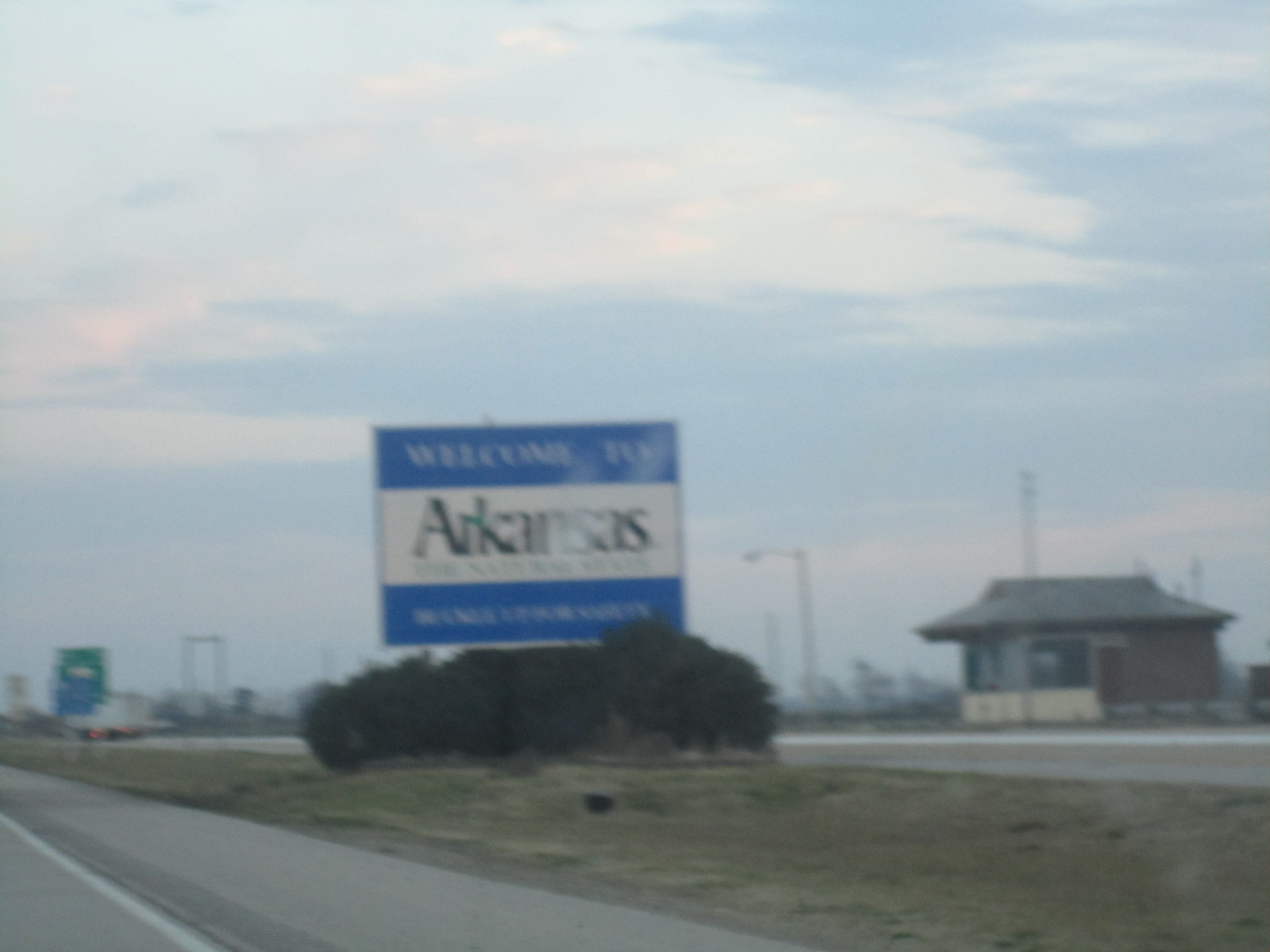The image captures a slightly out-of-focus scene from a roadside area near an entranceway, possibly into a state or a rest stop. Dominated by a mostly blue and white sky with hints of pinkish pastel colors, suggesting it could be sunrise or sunset, the photograph prominently features a large sign that says "Welcome to Arkansas." This rectangular sign, blue at the top and bottom with a white strip in the middle containing the text, is positioned on a grassy median strip accompanied by a small green bush at its base. To the left, a partially visible macadam road with a white line marking its edge runs from the bottom left corner upwards. On the right, the structure resembling a weigh station or rest stop office is visible, characterized by its simple one-story design with a greenish roof and glass front. Additional elements in the scene include various road signs in the background, with indistinct green and blue freeway signs above the left corner and a blurred white trailer from a big truck in the distance. Light poles and other signs can also be seen around the weigh station building. The overall mood of the photograph, despite its blurriness, is well-lit and vividly captures the outdoor scene.